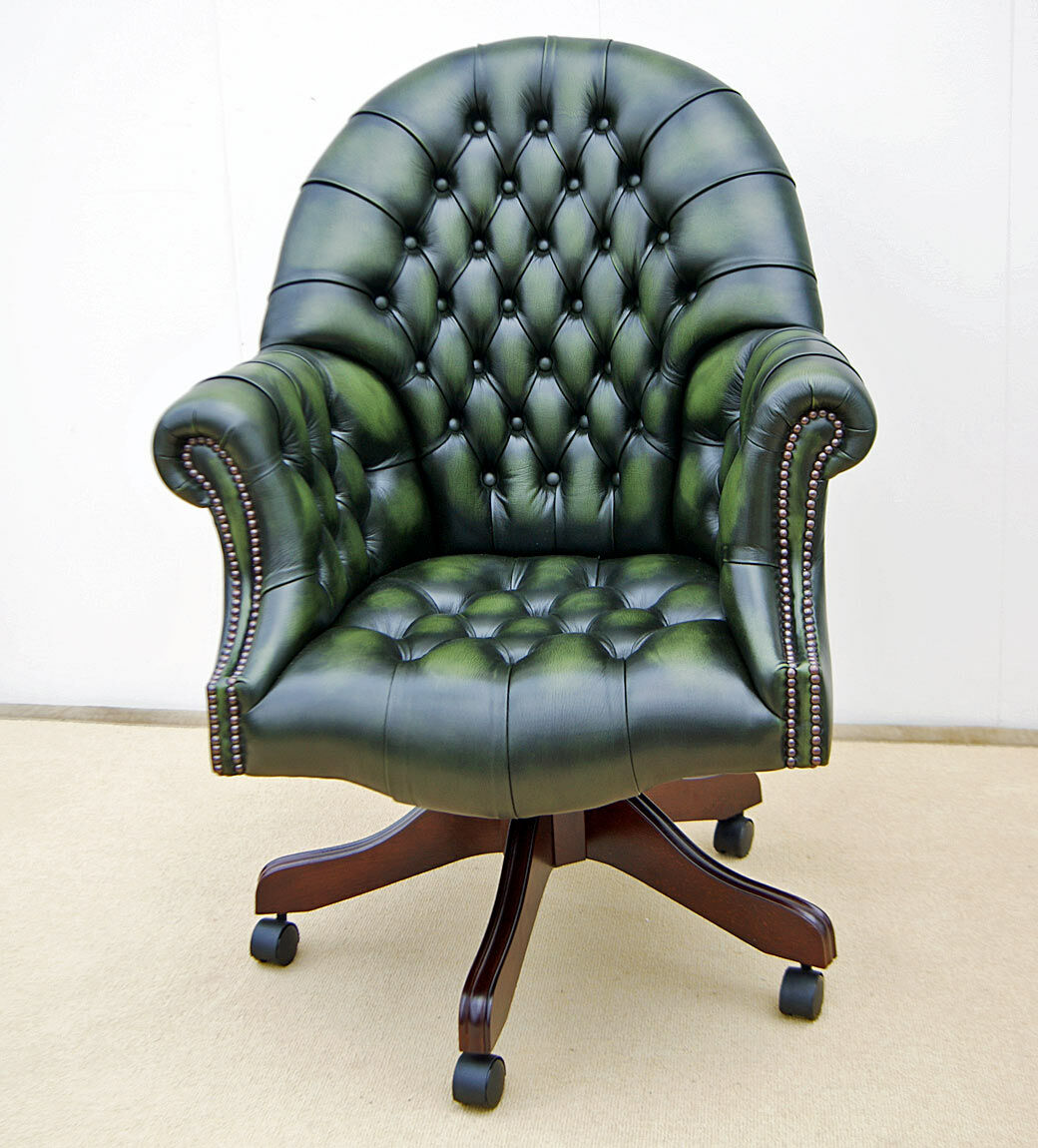In the image, we see a distinctive office-style rolling chair positioned on a light tan floor against a backdrop featuring a gradient wall that transitions from light gray on the right to whitish on the left. The wall is accented by a thin brown baseboard running along its length. The chair, facing the camera, is a mix of sophisticated design and vibrant color. It boasts a dark emerald green leather upholstery with lighter green accents, reminiscent of avocado or dark lime hues. The high, curved back and thick seat are adorned with multiple buttons arranged in a diamond pattern, adding to its designer appeal. The high arms of the chair also feature decorative embellishments. The chair’s base is star-shaped, brown in color, and supported by five black wheels, each attached to legs that splay out like wooden coat hangers. Despite appearing somewhat like a recliner, the chair lacks any reclining functionality. Its glossy, smooth texture and detailed craftsmanship make it stand out as not just a functional piece but also a statement of style.